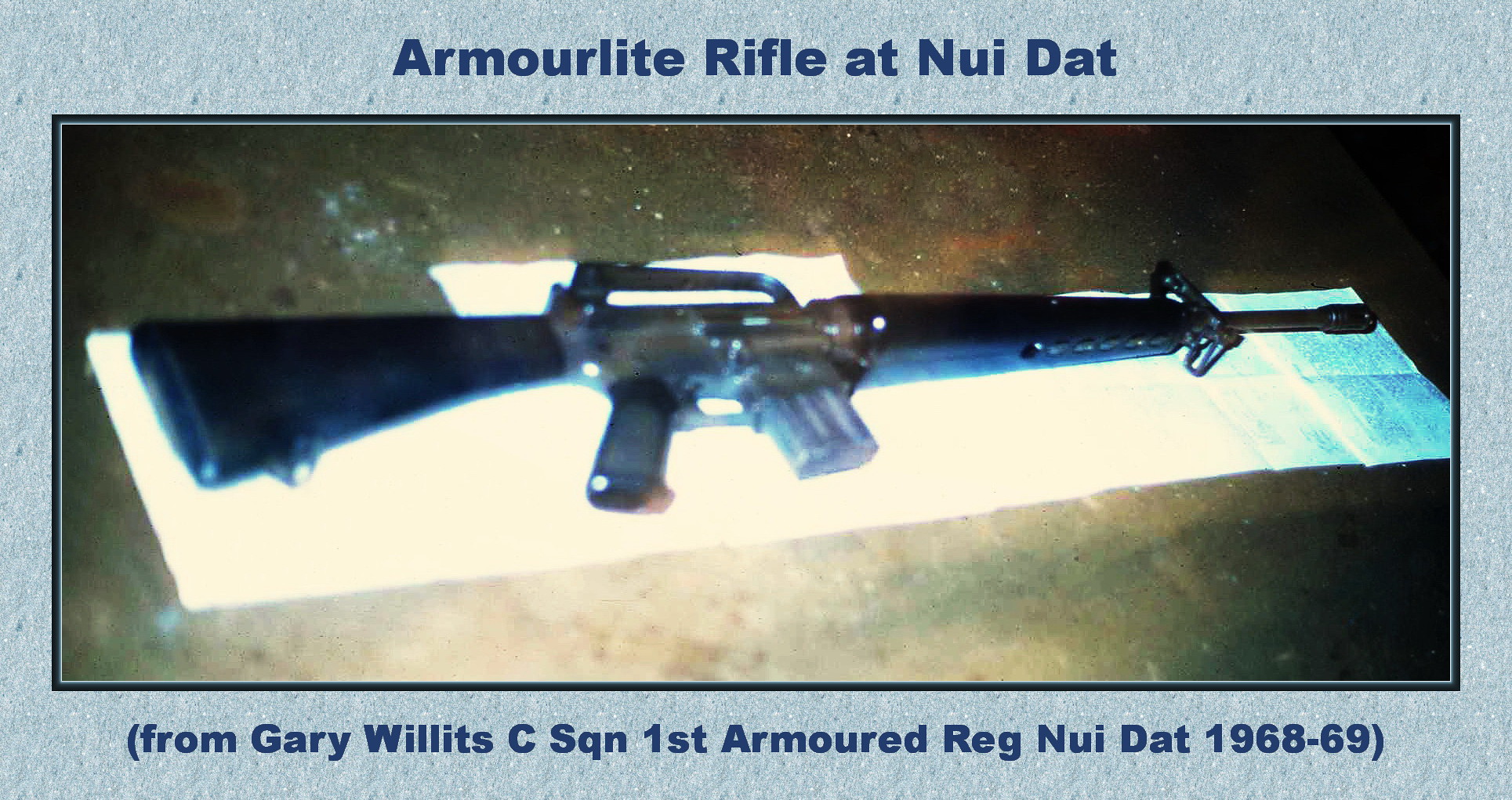The picture is a mounted photograph of a black semi-automatic rifle, specifically labeled as an "ArmaLite Rifle at Nui Dat." The rifle is positioned horizontally with the barrel facing the right and the shoulder rest on the left. It's laying on a white cloth, which sits atop a table featuring a dark, marbled texture with various colors. This table appears to be lit from underneath, giving a distinctive appearance.

The photograph is framed with a light black border and mounted on a textured powder blue background. Dark blue text at the top of the mount reads, "ArmaLite Rifle at Nui Dat," while text at the bottom states, "From Gary Willits, C SQN, First Armored Reg, Nui Dat, 1968-69." This suggests the rifle has historical significance, likely related to Gary Willits' military service during that period.